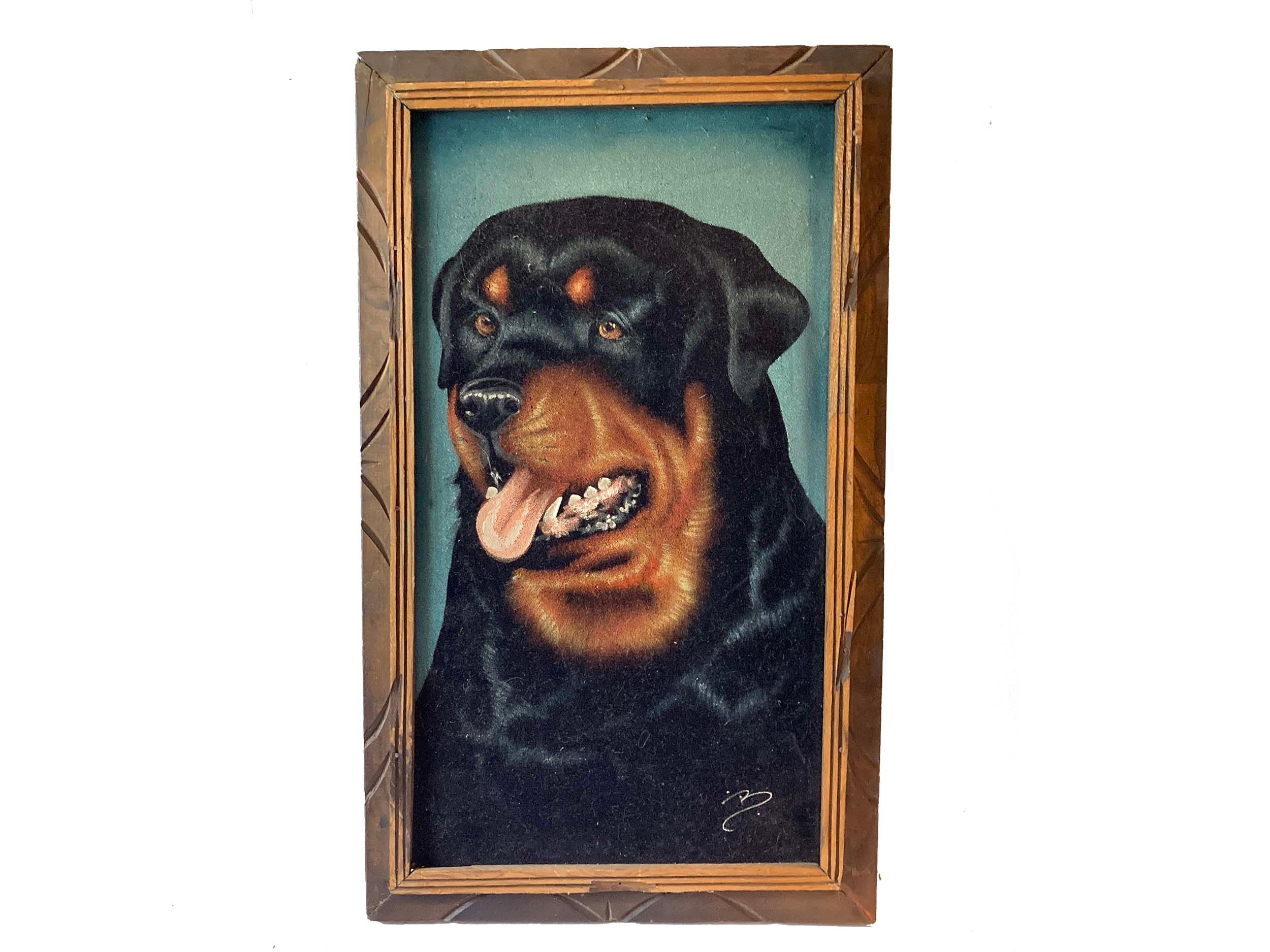The image features a detailed painting of a Rottweiler set against a light green background. The dog is depicted with a black coat featuring distinct brown areas around the muzzle, jaw, neck, and above the eyes. The Rottweiler’s head and neck are prominently displayed, with the neck appearing thick and the black fur looking remarkably shiny. The dog has its mouth open, showcasing its sharp teeth and pink tongue. Notably, the positioning of the mouth seems slightly off, appearing larger and somewhat detached from the head. Surrounding the painting is a brown wooden frame with intricate ridges along the borders. An inner frame with a striped wooden pattern adds depth to the presentation. The artist’s signature, resembling the letter 'B,' is signed at the bottom right corner of the painting.